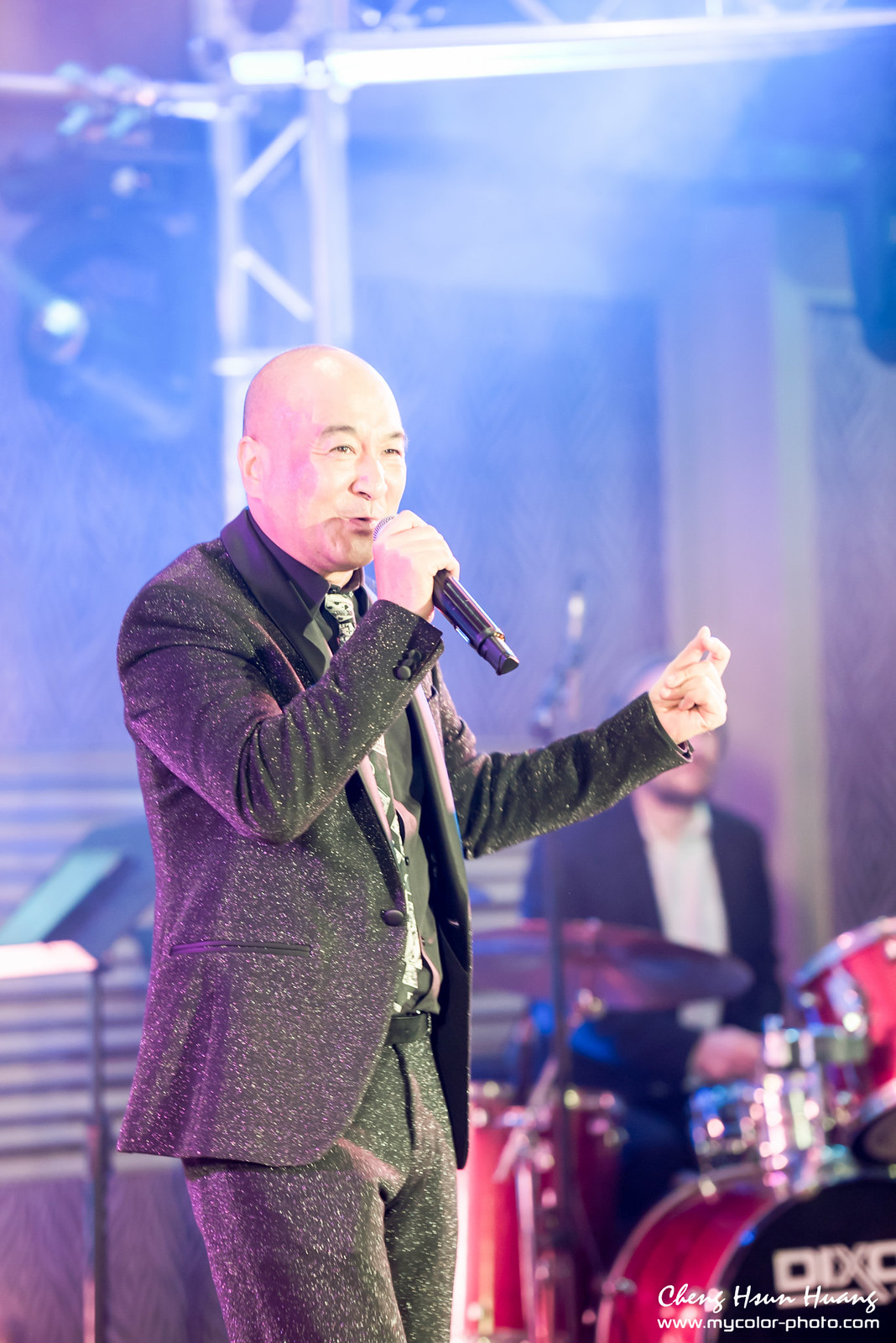The image captures the vibrant atmosphere of a live musical concert. In the background, the stage is brightly illuminated with blue lighting, accentuating the striking frames and blurred silhouettes of musical instruments, including a prominent red drum set. The drummer, dressed sharply in a black suit, black coat, and white shirt, can be seen behind the drums. 

Dominating the center of the image is the main artist, a bald, fair-skinned male who appears to be of Asian descent. He is impeccably dressed in a black blazer, black pants, and a black shirt, complemented by a stylish designer tie. Engaging with the audience, he is captured mid-song, holding a microphone in his right hand while snapping the fingers of his left hand in rhythm.

At the bottom right corner of the image, the words "Chang Soon Hwang, www.mycolor-photo.com" are visible, likely indicating the photographer and source of the image.